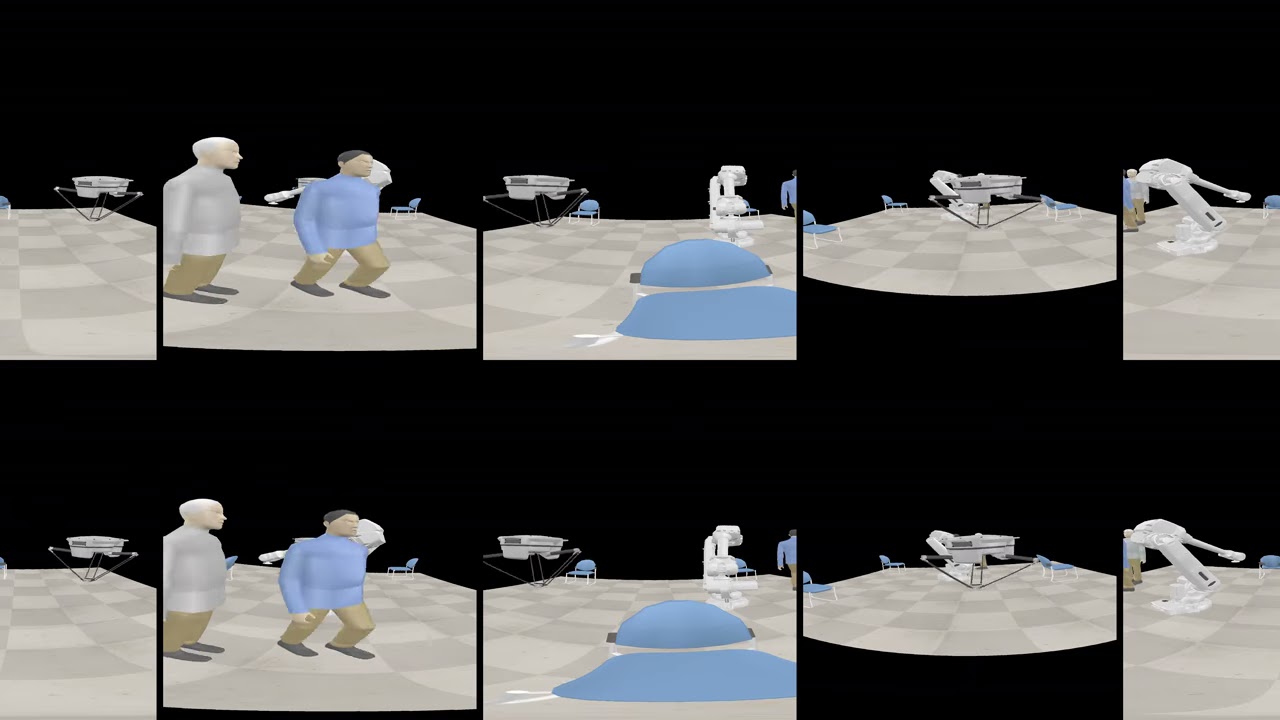The image depicts a series of animated segments arranged in two rows of five panels each, against a black background. The panels appear to represent a step-by-step procedural guide or a virtual reality program. Each panel is framed in a fisheye lens style, providing a slightly distorted yet detailed view of the scenes. The main colors within the panels are tan, white, blue, and black. 

Several elements are repeated across the panels:

1. **Robotic and Human Figures**: Both rows contain images featuring two individuals - one wearing a white shirt with tan pants and the other a blue shirt with tan pants, suggesting uniformity. They are depicted either standing or walking, with chairs and some machinery in the background. 

2. **Machinery and Apparatus**: There is a machine on a stand, prominently shown in the first and fourth panels, with the fourth offering a close-up view. Additionally, different robotic elements are present, including one that resembles a rabbit and another half-dome shaped blue object on the floor.

3. **Consistent Environment**: The environment in each panel maintains a consistent floor pattern of light and dark gray tiles, enhancing the computerized or virtual atmosphere. The floor and machinery are in contrast with the black background.

4. **Miscellaneous Objects**: A blue cloth-like object and a blue dome-shaped apparatus are seen in various panels, indicating part of a procedural setup or environmental detail.

Overall, the image provides a detailed and intricate look at a technological or virtual setup, featuring repeated elements such as robots, machinery, and human figures, all set against a uniform patterned floor and a stark black backdrop.